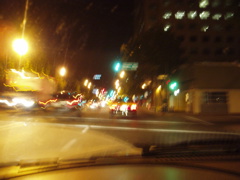The image captures an urban night scene from the inside of a car at an intersection, evidenced by the visible lower portion of the windshield wipers. The traffic light ahead shines green, accompanied by a green street sign. Although the image is small and details are somewhat unclear, the intersection is discernible with a few cars visible on the road, marked by their red taillights. To the left, there's a yellow illumination, likely from a lamppost. In the upper right corner, a towering skyscraper, adorned with numerous windows emitting white light, looms over the scene. Closer to the ground on the right, another building with a door is partially visible. The black sky indicates it is night time, adding to the city’s illuminated atmosphere.